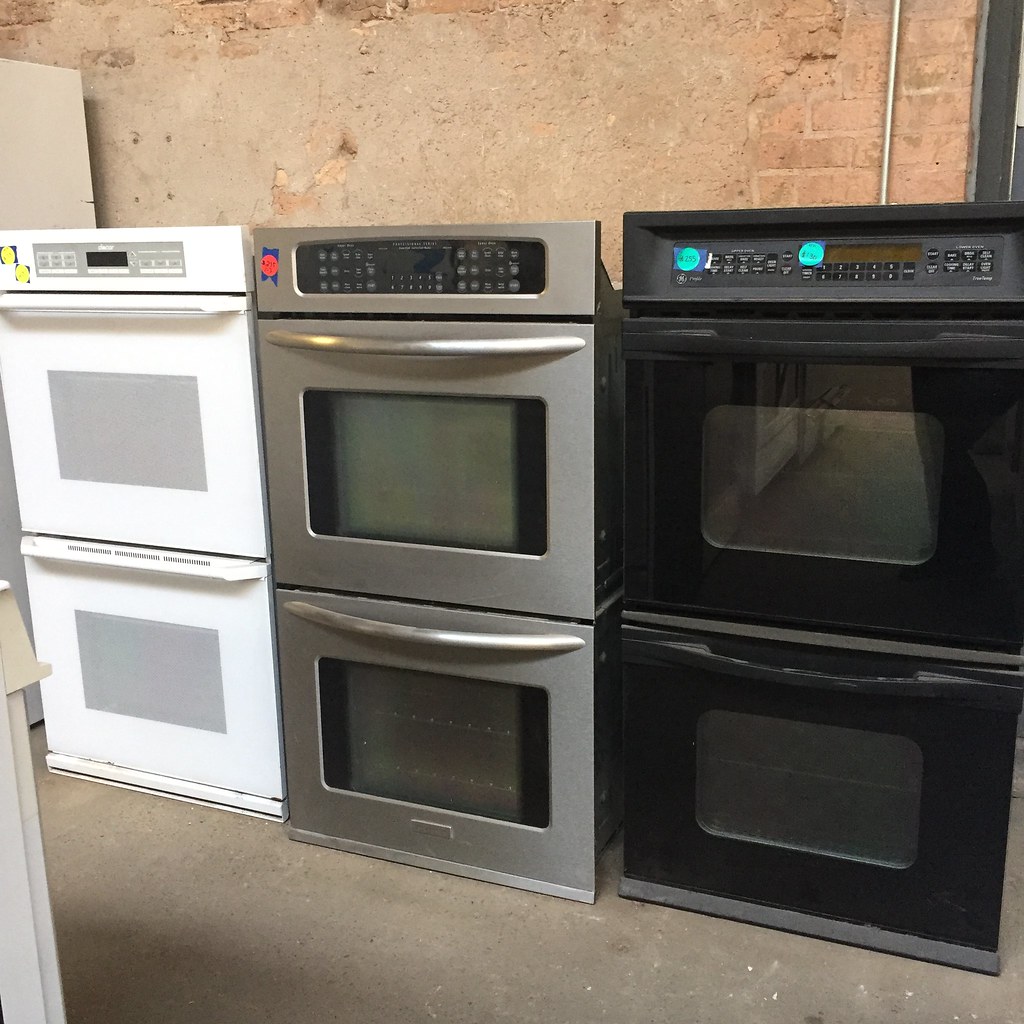This photograph, taken in a houseware store specializing in appliances, features a display of three double ovens arranged diagonally from left to right. The ovens are stacked, with each set comprising an upper and lower oven. On the far left, there is a white and gray oven with two yellow and blue stickers on its left side. The middle oven is primarily stainless steel with gray and black hues and bears a red and blue sticker on its left side. To the right, the all-black oven is adorned with bright green stickers showing partial numbers "130" and "255". Each oven has two doors with windows allowing visibility inside. All units are digital, though the specific numbers or letters on the buttons are unclear. The appliances are set against a backdrop of a worn reddish-brown brick wall, and the floor beneath them is a shiny, slightly dirty gray concrete.